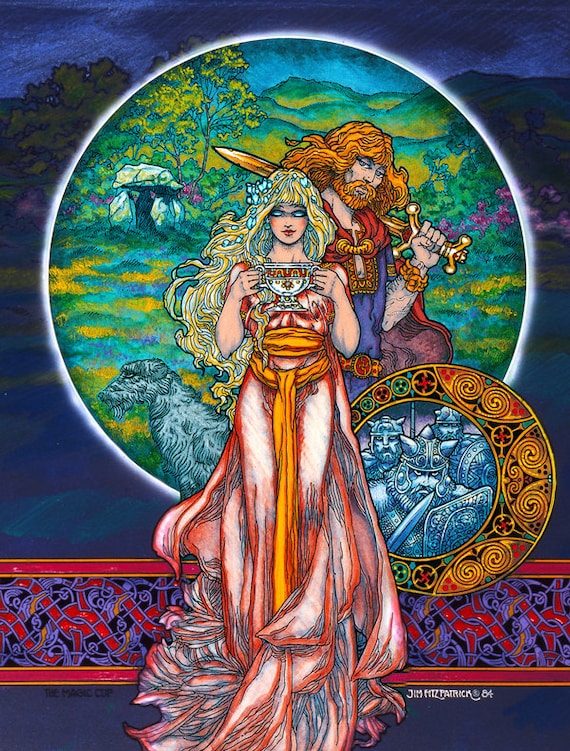This artwork titled "The Magic Cup" is a detailed illustration with a dark, mystical background featuring a dimly lit forest and silhouetted trees. On the left is a striking tree, while to the right stands an imposing mountain. The central focus is an illuminated circle that contrasts sharply with the surrounding darkness, filled with vibrant greenery and a pastoral scene.

Inside this circle stands a majestic woman with long, flowing blonde hair adorned with blue particles or flowers. She wears a flowy pink and blue dress with a yellow waistband extending down the front. Her blue, pupil-less eyes lend her an ethereal presence. She holds a silver chalice with both hands close to her neck, suggesting a divine or ritualistic significance. By her left side is an Irish wolfhound, adding to the fantastical ambiance.

Behind her is a Nordic warrior, distinguished by his long red hair and beard, clothed in a purple tunic with a red cape. Wielding a large, golden sword over his shoulder, he stands protectively. Behind him, the miniature Stonehenge suggests ancient mysticism and further deepens the scene's historical richness.

In the upper right of the circular area, another, smaller ring depicts a battle between warriors, surrounded by decorative Norse elements in yellow, green, and gold. At the bottom, a band of intricate Nordic patterns in red, gold, and purple adds an artistic border to the piece.

The artwork, which resembles stained glass with its vibrant colors and outlined style, is signed "Jim Fitzpatrick '84" in the bottom region. This signature is placed above a decorative band that stretches across the bottom of the image, further enriching the scene's cultural tapestry.